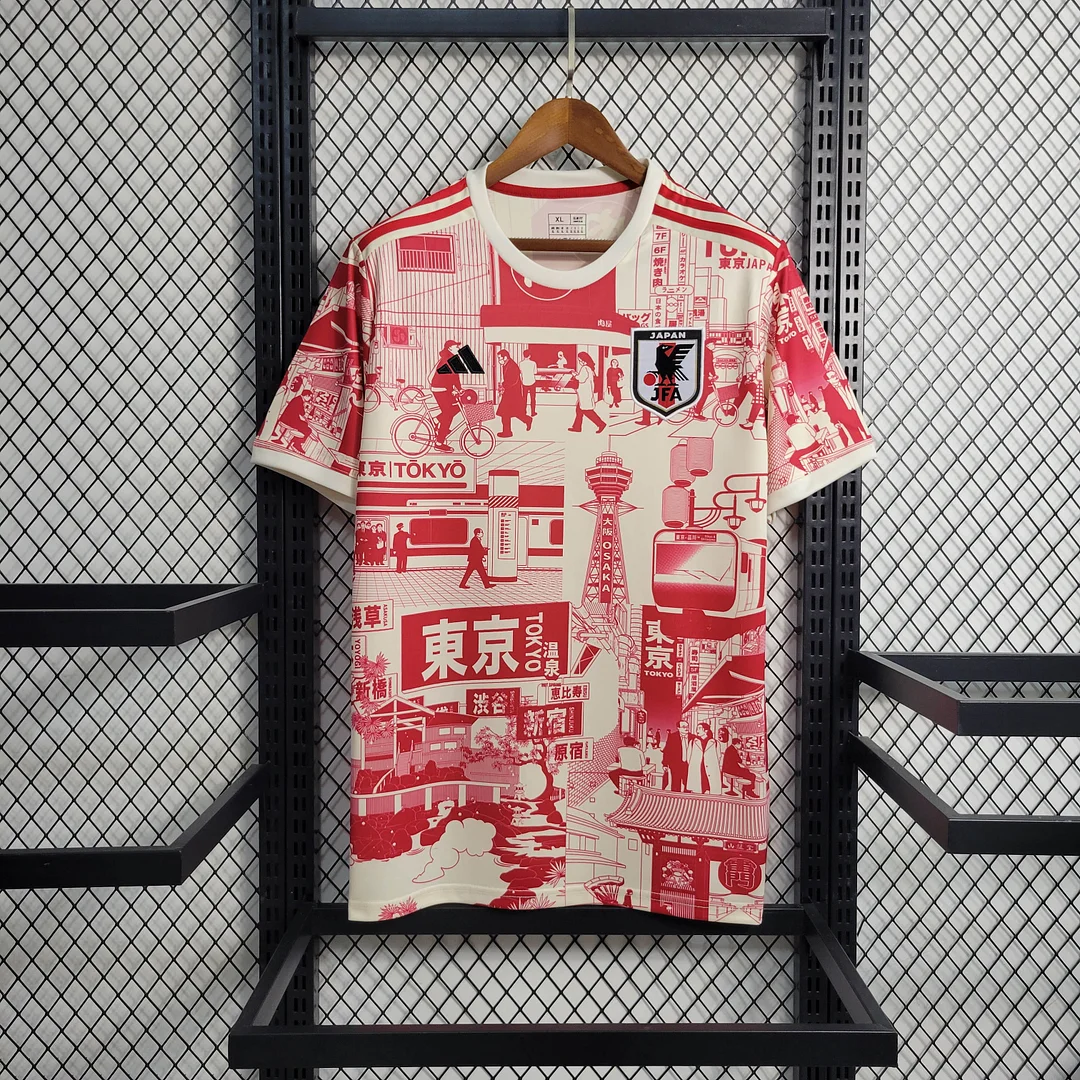This image features a high-definition, up-close photograph of a red and white Adidas jersey displayed on a wooden coat hanger. The background consists of a black chain-link fence-like mesh with metal bars, suggesting an organizational layout, possibly within someone's closet. The jersey, which is the main focus of the image, is predominantly red with a white backdrop and adorned with various Japanese-themed graphics. Detailed imagery on the shirt includes scenes from Tokyo, such as people walking on sidewalks, riding bicycles, and standing in subway stations with "Tokyo" and "Osaka" written in various places. The Adidas logo is visible on the right side of the chest, while on the left side, the emblem features the Japan Football Association (JFA) logo, which includes an eagle motif. The jersey is marked as an XL size. The design also incorporates the classic Adidas stripes running down the shoulders, enhancing the overall aesthetic of this visually striking shirt.